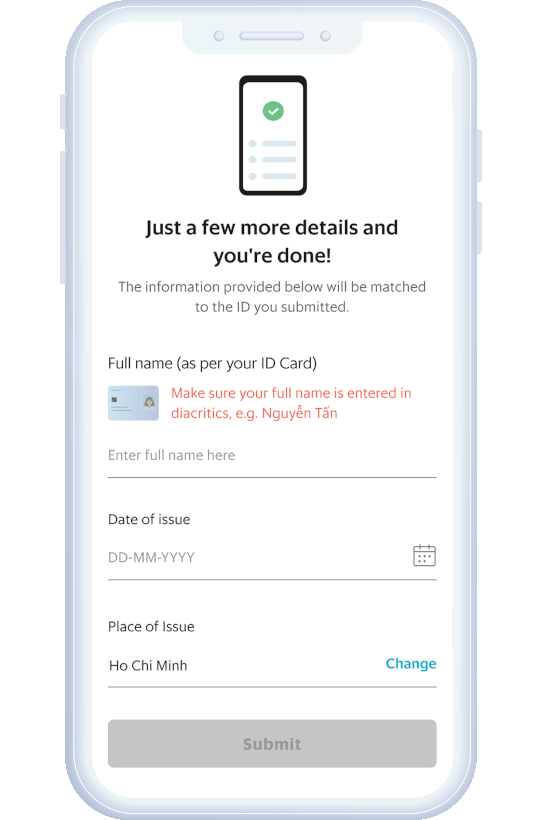In the image, a rendered cell phone screen displays a registration form for an ID card application. At the center of the screen, an app interface shows a message: "Just a few more details and you're done." Below that, in smaller text, it reads: "The information provided below will be matched to the ID you've submitted."

Further down, there is a field labeled "Full Name" with a hint in parentheses: "as per your ID card." The instruction in red font below advises, "Make sure your full name is entered in diacritics such as 'N-g-u-y-e-n-T-a-n.'"

Next, there is an input space for the name. Below this field, another label reads "Date Issued" with a specified format instruction: "dd/mm/yyyy." Following this is another field labeled "Place of Issue" which has been auto-filled with "Ho Chi Minh." To the right, there is an option to "Change" this information.

The form depicted in this app appears to be a sample pulled from a website, illustrating the required information and the expected format for filling out an ID card application. Key instructions include entering the full name with diacritics and using the day/month/year format for the date. Diacritics refer to the use of accent marks and other special characters in names.